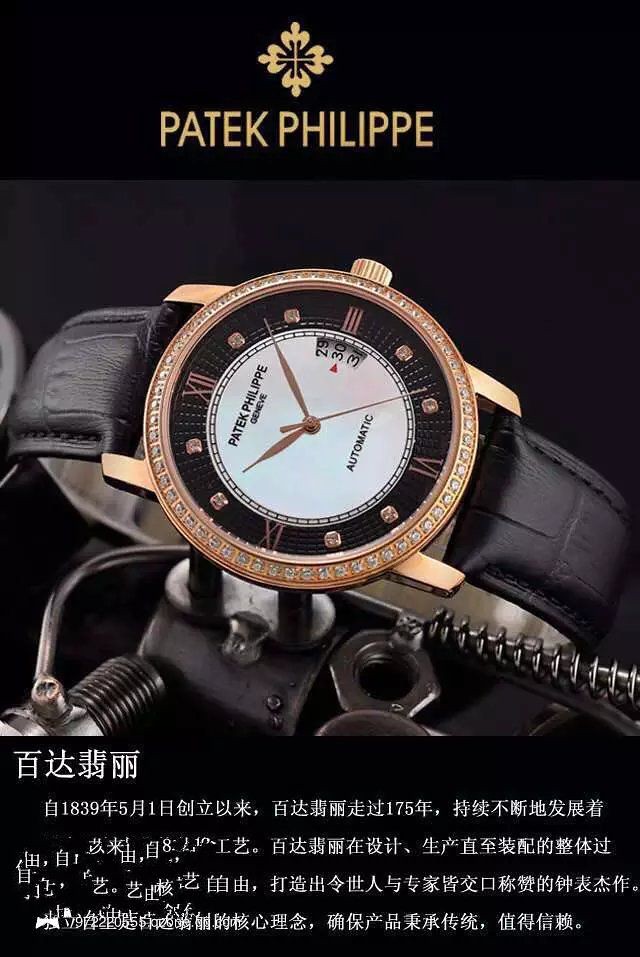This advertisement photograph showcases an exquisite men's watch by Patek Philippe, prominently labeled at the top of the image in a gold font on a black background, with their iconic cross-like logo. The watch itself is a masterpiece of luxury, featuring a high-quality black leather strap and a stunning 24-karat gold bezel, adorned with small, intricately placed diamonds. The dial is primarily white, set against a black backdrop that houses gold hour and minute hands and a red-tipped date indicator pointing to the 30th. Roman numerals for 12, 3, 6, and 9 are visible, while the remaining numerals are marked by sparkling jewels. The face also displays "Patek Philippe" and "Geneva" at the top left, and "Automatic" near the 3 o'clock position. This elegant timepiece is presented horizontally against a black background, resting among industrial elements such as nuts, bolts, and possibly gears, to emphasize a striking contrast between industrial ruggedness and refined beauty. At the bottom, the image features Asian text, suggesting the advertisement targets an Asian market, although the specific language is unclear.